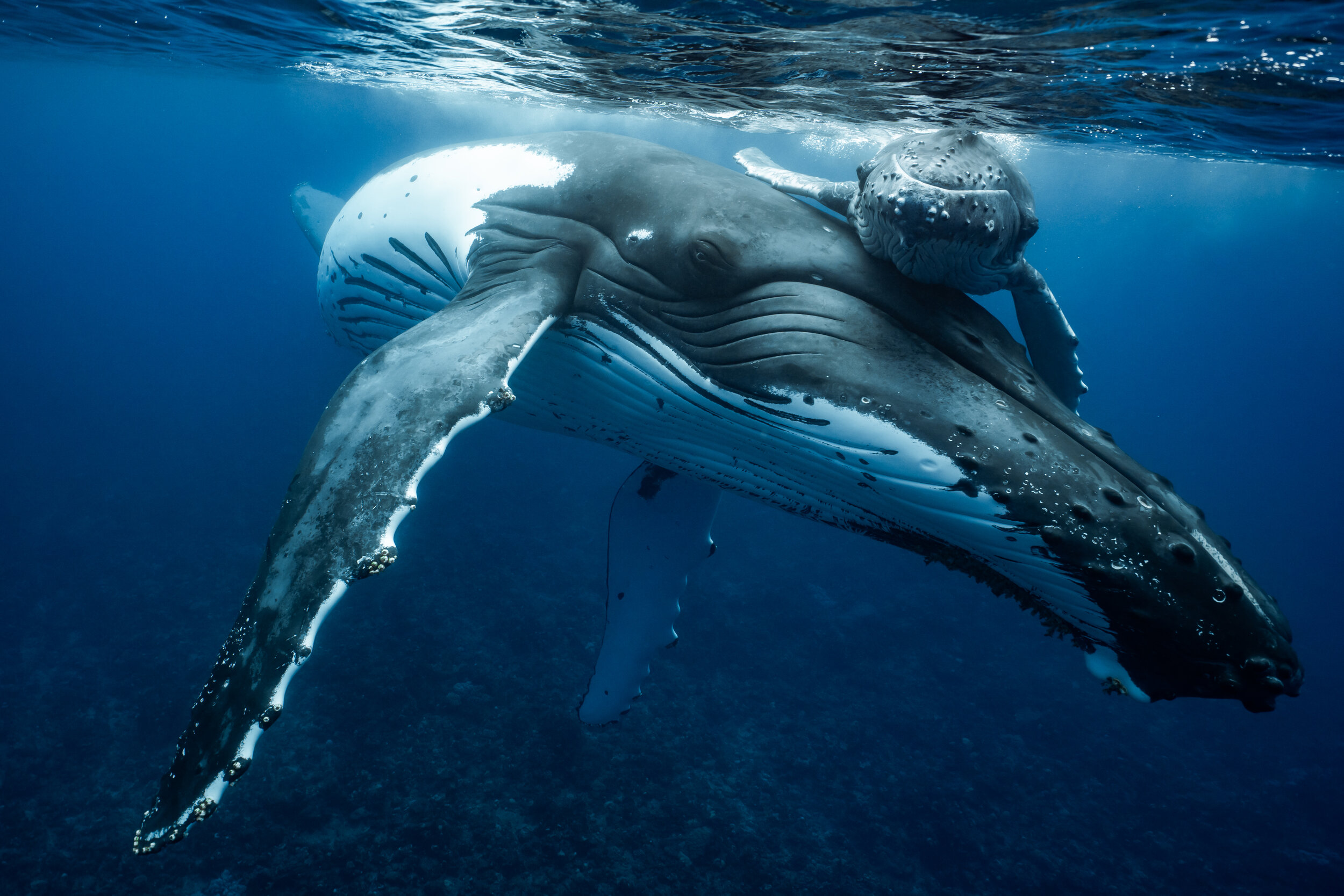This is a realistic underwater photograph, horizontally oriented, depicting an intimate moment between an adult whale and a baby whale. Both whales, colored grayish blue on top and white on the bottom, are seen underwater, appearing to touch faces as if bonding or hugging in a serene display of affection. The image captures them facing the camera, showcasing their front faces and fins while their backs remain unseen. 

The water is a vivid blue, perhaps 20 to 30 feet deep, with some white reflections indicating sunlight filtering in from the surface, which is visible in the background. The sea floor, located at the bottom of the image, features algae, rocks, and small plants, adding depth and natural environment to the scene. The interaction suggests a close relationship, possibly parent and offspring, as they slowly swim near the surface of the ocean.